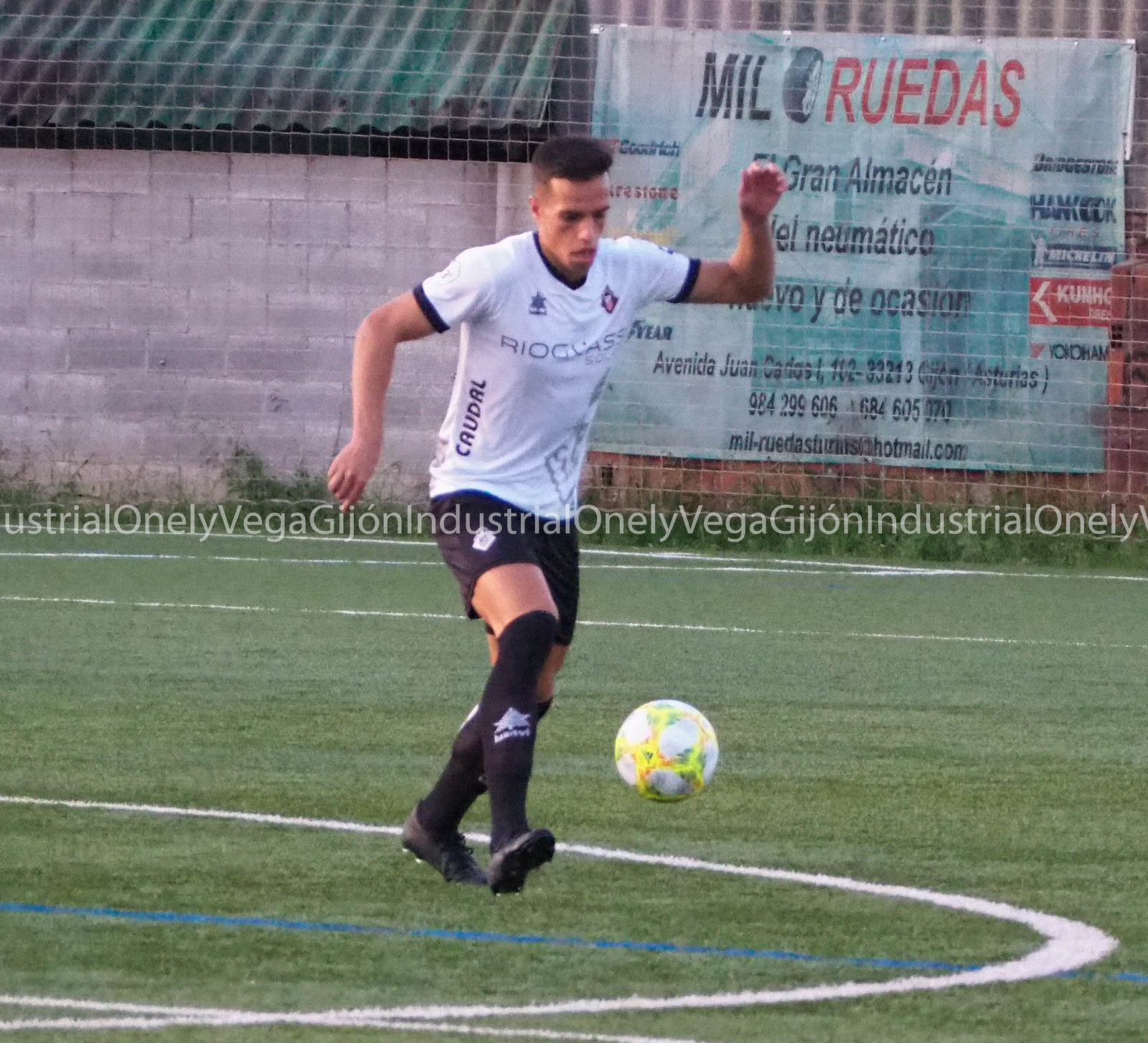The image features a focused soccer player in mid-action on a green turf field with white and blue painted stripes. He is positioned in the center of the field, wearing a white jersey with black lettering, black shorts, black long socks, and black cleats. The young athlete, who has short dark hair, is seen kicking a white and yellow soccer ball with his arms raised, eyes fixated on the ball. In the background, there is a brick wall with a corrugated tin roof building and a large white banner displaying various tire brands such as Yokohama, Bridgestone, and Michelin, along with the words "Mill Rui does" and images related to tires. The banner is mounted on a fence, adding depth to the scene, which suggests it might be set in a Latin American or Latin European country. The sun is shining, indicating it is daytime.